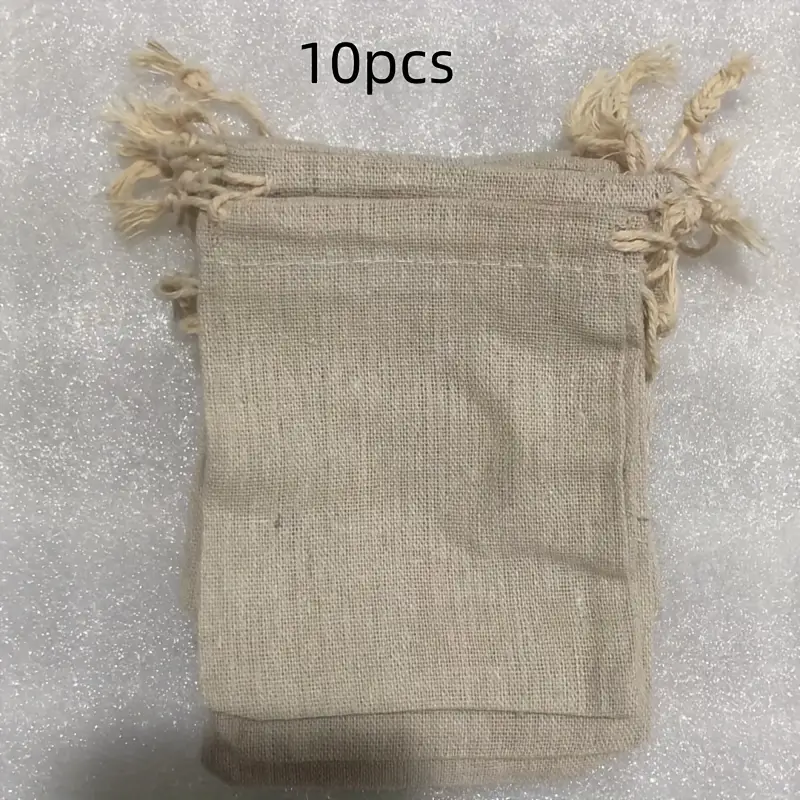This image features an advertisement showcasing a pile of 10 small brown satchels, prominently labeled with "10 PCS" in black text at the top center. These satchels are crafted from a tan-colored, coarse canvas material, often mistaken for burlap or linen, showcasing a rustic appearance with visible space between the threads. Each satchel is rectangular and features a drawstring closure made of twine that is stitched and knotted at both ends, which can be pulled to secure the contents inside. The background of the image is a speckled white-gray surface, adding a clean and contrasting backdrop to the earthy tones of the bags. The satchels, slightly misaligned in the stack, hint at the texture and flexibility of the material, making them ideal for storing small collections such as rocks, marbles, or coins.